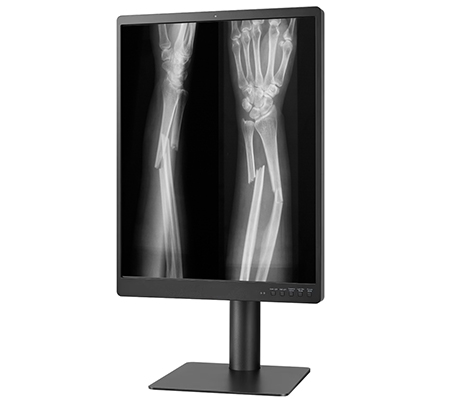The image displays a modern, rectangular LCD x-ray monitor, predominantly black with a black screen, standing against a white background. The sleek monitor, taller than it is wide, features a broad cylindrical stand and a thin rectangular base. In the bottom right corner of the monitor's border, five circular buttons with indistinct white text are visible. On the screen, there are two x-ray images of a right arm, revealing a severe and painful fracture. The x-rays exhibit both a top view and a side view, depicting a complete break in the ulna (the smaller bone) and a bowed, cracked radius (the larger bone). The broken bones in both views suggest a need for surgery and pins to repair the fractures.